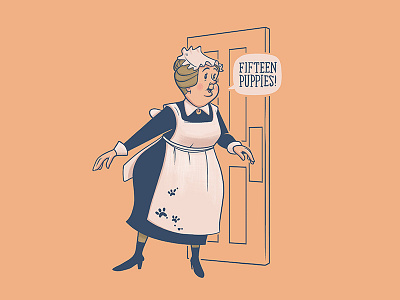The image is an animated drawing featuring a maid reminiscent of the character from "101 Dalmatians." The background is a soft peach or light orange color, providing a smooth, solid contrast to the outlined elements. In the center of the image is a door, drawn simply with black outlines, including a handle and four rectangular panels, though partially obscured by the maid. The maid is an older, heavyset woman with her hair pulled back into a bun colored in a brownish-gold hue. She is dressed in a classic maid's outfit—a navy blue dress with a white collar and cuffs, white apron tied in a bow at the back, and matching navy boot-like shoes. On the apron, there are notable navy paw prints on one corner. She wears a traditional white maid cap, and her face shows a surprised expression. A speech bubble, drawn in blue with a white background, contains the text "15 puppies," capturing a memorable scene from the movie. The minimalistic and stylistic elements, along with her iconic statement, suggest that this image might be designed for a product like a t-shirt.